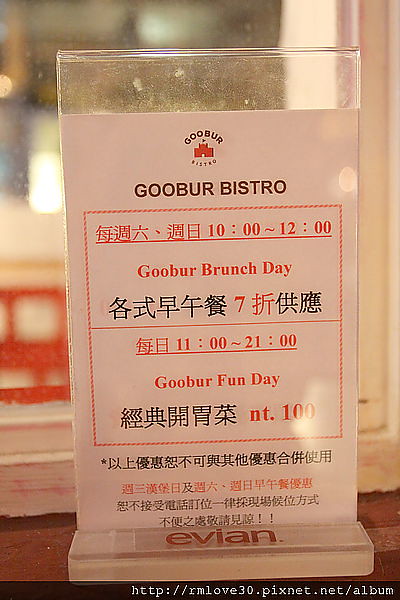This color photograph, taken in portrait orientation, features a clear plastic restaurant table placard with a white piece of paper inserted inside. The paper, printed in both red and black fonts, displays multiple details about Goober Bistro. At the top, there's a logo with a red castle and the text "Goober Bistro, G-O-O-B-U-R." Beneath the logo, a range of hours is listed along with events titled "Goober Brunch Day" (10 to 12) and "Goober Fun Day" (11 to 21), followed by "NT100". The text also includes various characters in an Asian language, likely Chinese or Japanese, which are interspersed between the English phrases. The base of the placard prominently features the Evian logo in red script. The setup is stationed on a brown surface placed in front of a window that opens to a blurry outdoor scene. Across the bottom of the image is a URL: http://rmlove30.pixnet.net.